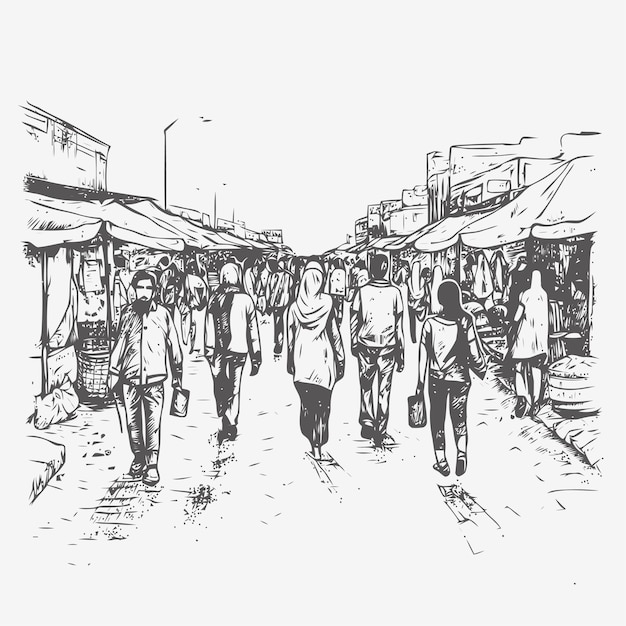The image is a detailed black and white, computer-generated pen and ink style drawing of a bustling marketplace, likely set in the Middle East, as suggested by the traditional dress of the people. The background is a light grayish-white. The scene is set on a cobblestone street lined with vendor stalls on both sides, covered by canopies and awnings, with various indistinct wares including barrels and baskets. In the immediate foreground on the left is a man with a full dark beard, wearing a jacket, jeans, and sandals, holding a small bag in his left hand walking towards the viewer. Surrounding him are four other figures walking away, including women wearing headscarves and long tunic-style shirts with balloon pants, and one person carrying a purse. Small details, such as streetlights hanging above and the slightly elevated curbs at the edges of the cobblestone street, add depth and context to the vibrant market scene. The perspective of the image is slightly elevated, providing a comprehensive view of the crowd and the general hustle and bustle of the marketplace.